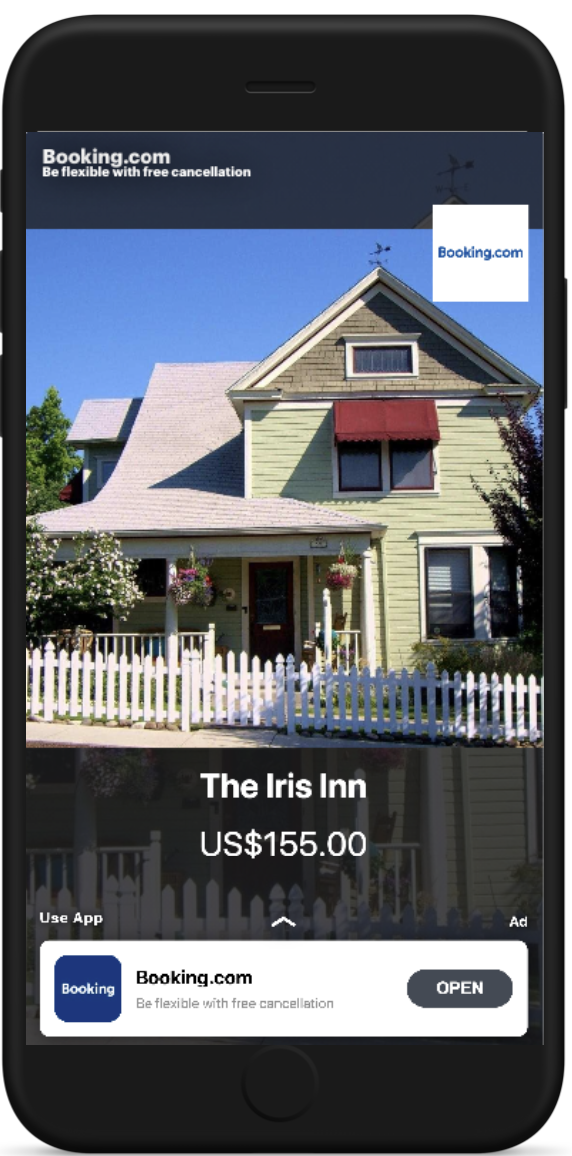The screenshot displays a phone screen featuring the Booking.com app. Dominating the right side of the screen is a white square with a blue "booking.com" logo. The image showcases a charming green house with a beige ceiling, adorned with a white picket fence and hanging plants on the porch. The house is surrounded by lush trees and bushes under a clear medium blue sky. The listing reads "The Iris Inn, US $155", and includes a prompt to "Use app" alongside a blue square with white text stating "booking". Additional text promotes flexibility with free cancellation, and there is a gray oval button with the word "open" in white.